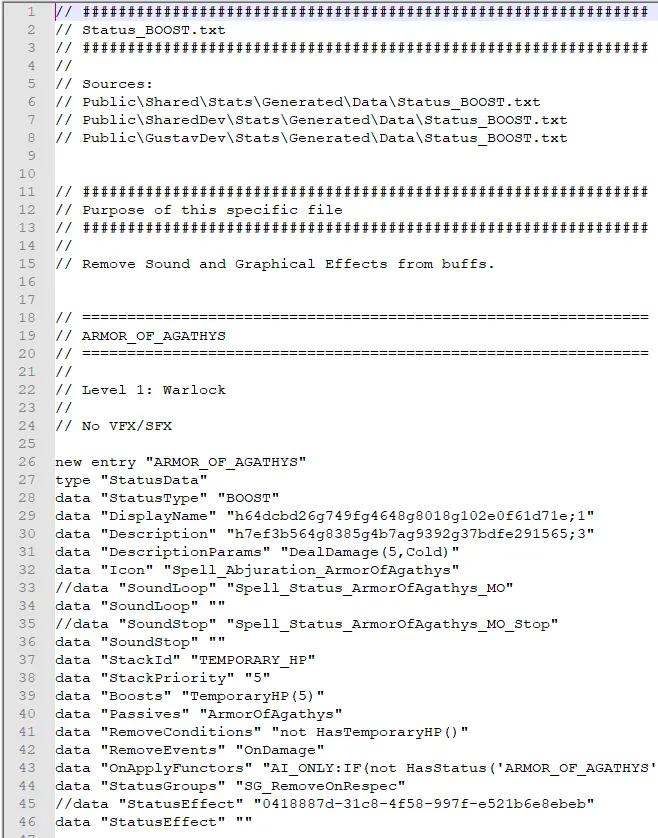The image displays a screen capture resembling a printed piece of paper from an old computer, with a white background. A very thin black line outlines the top and left borders of the image, suggesting that the border continues to the right and bottom, indicating this is only a portion of the complete image.

On the left side of the image runs a light gray column containing numbers sequentially listed from 1 to 46, with a partial visibility of the number 47, indicating more content beneath. Across the top of the image, a light gray or blue-gray bar spans horizontally. Within this bar, two backslashes (\\) are followed by a row of pound signs or hashtags (#) extending all the way across.

The numbered column starts with number 1 corresponding to the blue-gray bar with hashtags. Number 2 lists two backslashes with the entry "STATUS_BOOST.TXT" in all caps. The pattern continues along the left, with the column numbering entries related to backslashes and textual data. For instance, number 3 mirrors the first row with two backslashes followed by a row of hashtags.

The entries proceed as follows:
- Number 4: Two backslashes without additional text.
- Number 5: "Sources:"
- Number 6: "PUBLIC\\SHARED\\STATS\\GENERATED\\DATA\\STATUS_BOOST.TXT"
- Number 7: "PUBLIC\\SHARED\\DEV\\STATS\\GENERATED\\DATA\\STATUS_BOOST.TXT"

This pattern of coding or data paths continues with intermittent blank lines, denoted hashtags, and specific file designations.

Further into the list:
- Number 12: "Purpose of this specific file" framed by rows of hashtags on entries 11 and 13.
- Number 15: "Remove sound and graphical effects from buffs on" with an adjacent blank space.

By number 18, double lines created by equal signs (==) appear, with number 19 detailing "ARMOR_OF_AGATHYS" in caps, separated again by another double-line of equal signs.
- Number 22: "\\\\Level one: warlock", potentially indicating game programming language or script.

The document continues similarly, with a structured distribution of metadata, commands, and configurations, indicating that the image likely represents a snippet taken from a larger source code or script, possibly related to game development.